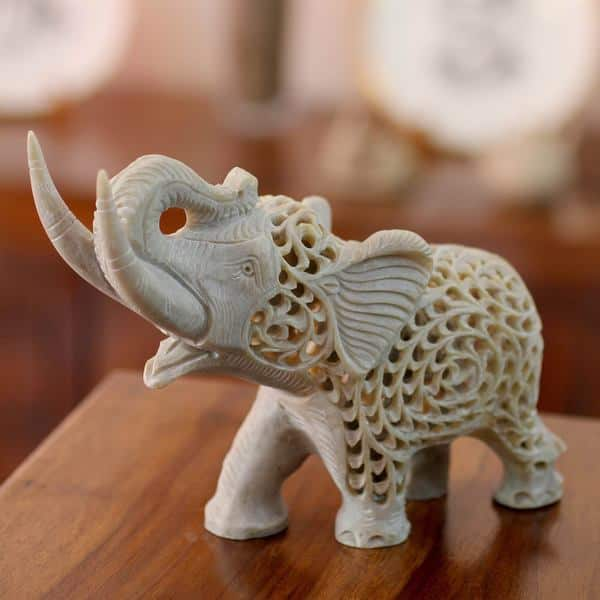This photo captures a detailed image of an intricately carved elephant figurine, which appears to be made from a white or ivory-like material, possibly ceramic, soapstone, or plastic. The elephant is positioned on a brown wooden table, and the background is blurred, revealing indistinct shapes that resemble white plates or other ornaments. The elephant’s two tusks extend forward, and its trunk is lifted and rests on its forehead, revealing an open mouth with visible tongue detail and distinct ears. The right side of the elephant is particularly notable for its decorative, curling designs and numerous holes, giving it a see-through, almost hollow appearance. This intricate detail allows light to pass through the sculpture, enhancing its artistic allure. Despite its beauty, there's an underlying hope that the material isn't actual ivory, juxtaposing the elegance of the art with ethical considerations.